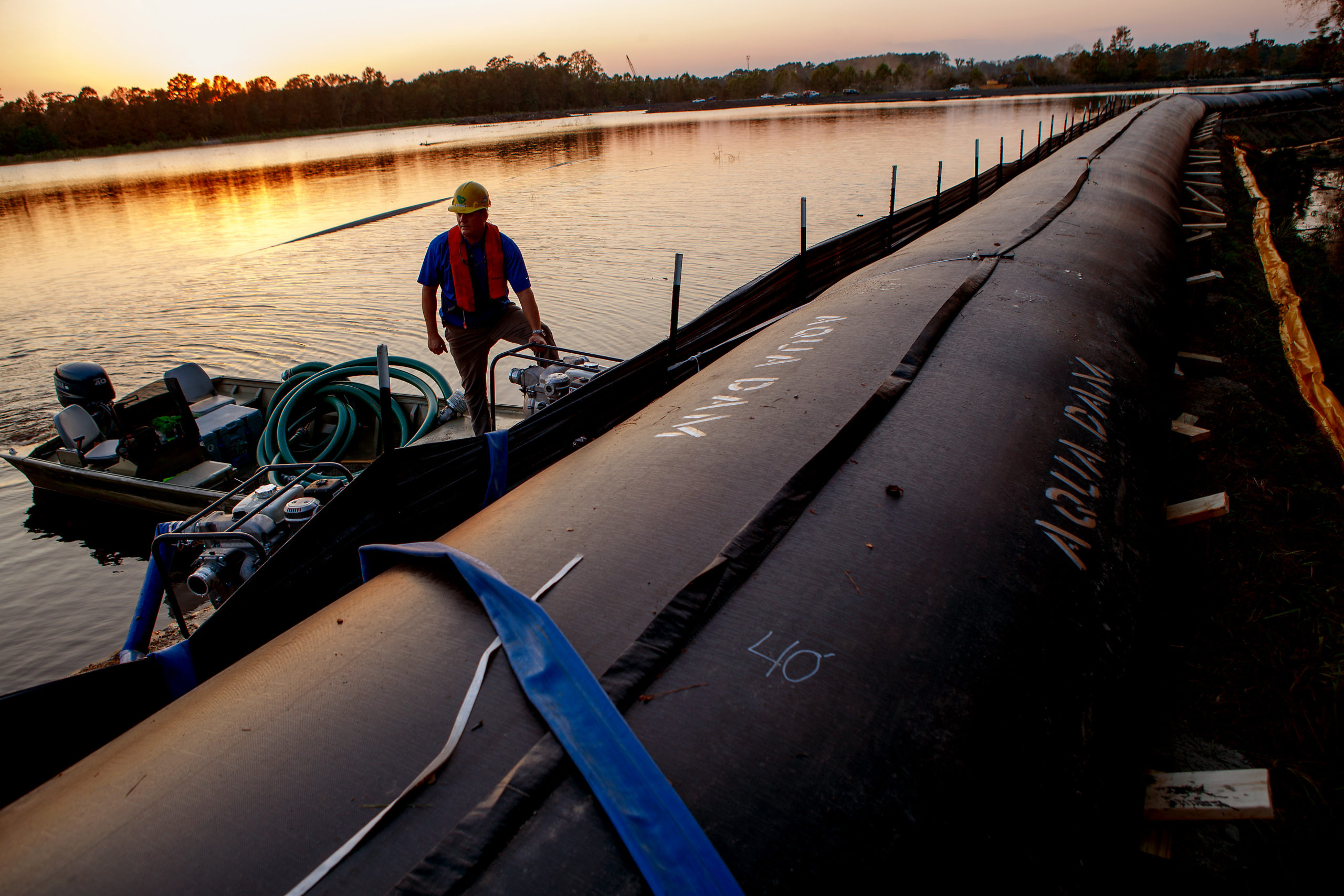The image depicts a sunset scene along a rural river, possibly in Mississippi or Louisiana. A long, inflatable tubular structure labeled "Aqua Dam" stretches diagonally across the water, its black surface reflecting the fading orange light of the setting sun. Trees line the riverbank, their dark silhouettes mirrored in the still water. A small boat is moored next to the Aqua Dam, with a man clad in a blue shirt, an orange vest, and a yellow hard hat straddling the boat and the dam. Nearby, various equipment including green hoses and small generators indicate ongoing work. The man appears to be engaged with the Aqua Dam on the lakeside, though his exact task remains unclear.